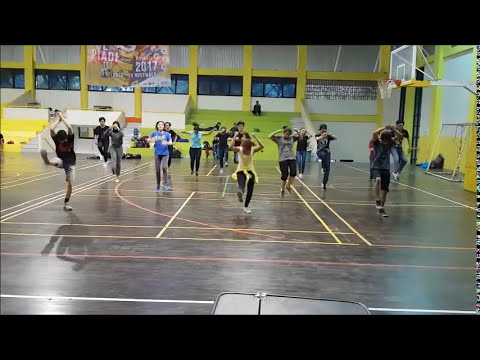The image depicts a gymnasium filled with middle school students engaged in what appears to be a dance or exercise class. The gym features clean, polished hardwood flooring marked with various colored lines—yellow, pink, and orange. On the right side, there's a basketball hoop, and in the background, bleachers in shades of green, yellow, and white are visible, with numerous windows above them. A small sign reading "Place 2017" is prominently displayed in front of the windows. The participants, wearing a variety of casual clothing such as leggings, t-shirts, and shorts, are following the lead of an individual at the front, who wears black pants and has a yellow shirt tied around their waist. This person, with arms raised, seems to be guiding the group through the activity. Some participants have their right leg extended up, showing variations in flexibility with some bending their knees while others maintain a straight leg. Additionally, a soccer or hockey goal net is visible on the right side, adding to the multipurpose nature of the gymnasium.